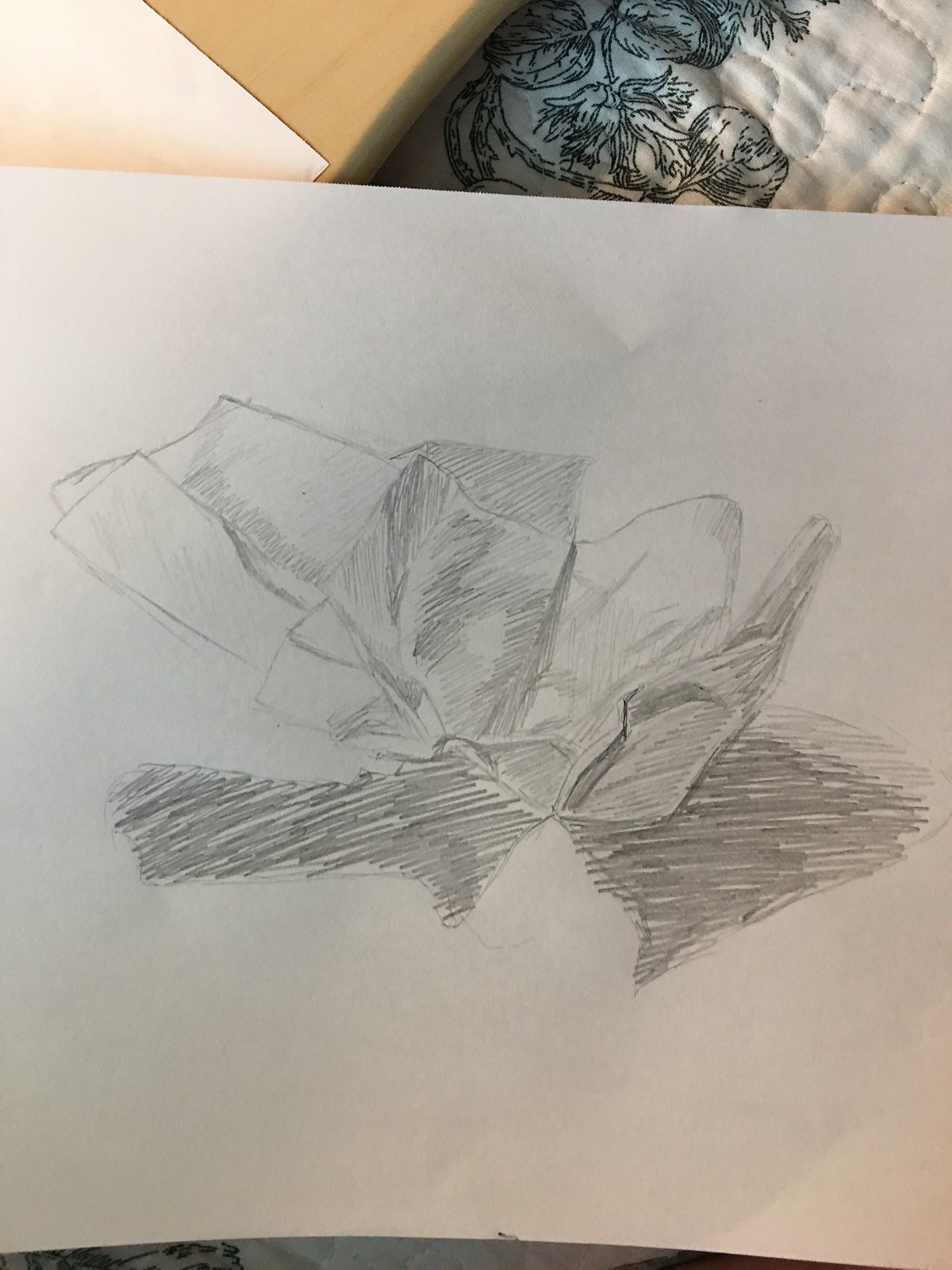This is a photograph of a vertical pencil drawing on a crinkled white sheet of paper. The drawing, which appears somewhat abstract and sketched quickly, consists of heavily and lightly shaded areas. The top part of the drawing features layers of what seem to be folded papers with varying degrees of shading, while at the bottom, there are fully shaded rectangular shapes, one to the left and another to the right, with the right one slightly larger. Near the top right corner of the sheet, vague flower-like ink images can be discerned. The background includes the corner of a light brown table and possibly a seat cushion with a floral pattern, adding context to the setting of the photograph. The entire composition suggests an intricate yet unclear subject, possibly a flower or crumpled papers, rendered with detailed pencil work.